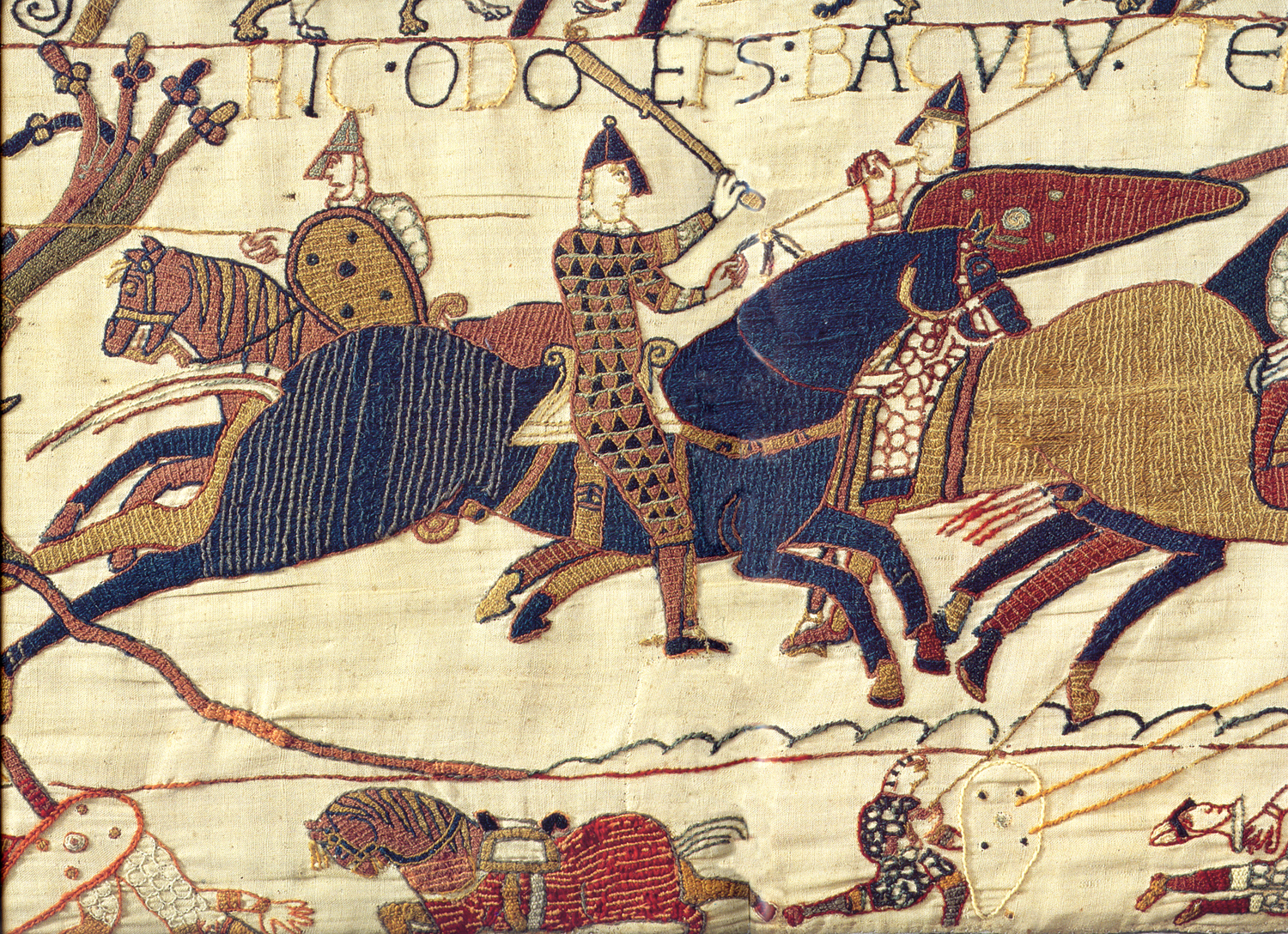This detailed rendering depicts a historical medieval battle scene, possibly an embroidery on a primitive ivory cloth, showcasing a vivid tapestry of armored knights engaged in combat. The knights, adorned in gold and navy blue armor, wield spears and shields of various hues, primarily red and yellow. They ride horses of differing shades, including black, brown, yellow, navy blue, gold, and bronze, with some horses sporting manes and others without. The chaotic battle unfolds with scenes of valor and agony: knights with arrows piercing their bodies, collapsing and clutching themselves amidst the fray. Above the intense melee, medieval text stretches across the image in gold and black lettering, spelling out "HICO DO EFS BACVL VTE," though the words appear fragmented or misspelled. The overall texture of the piece suggests that it could be made of fabric or be reminiscent of ancient cave paintings, firmly situating this artwork within a European medieval context.